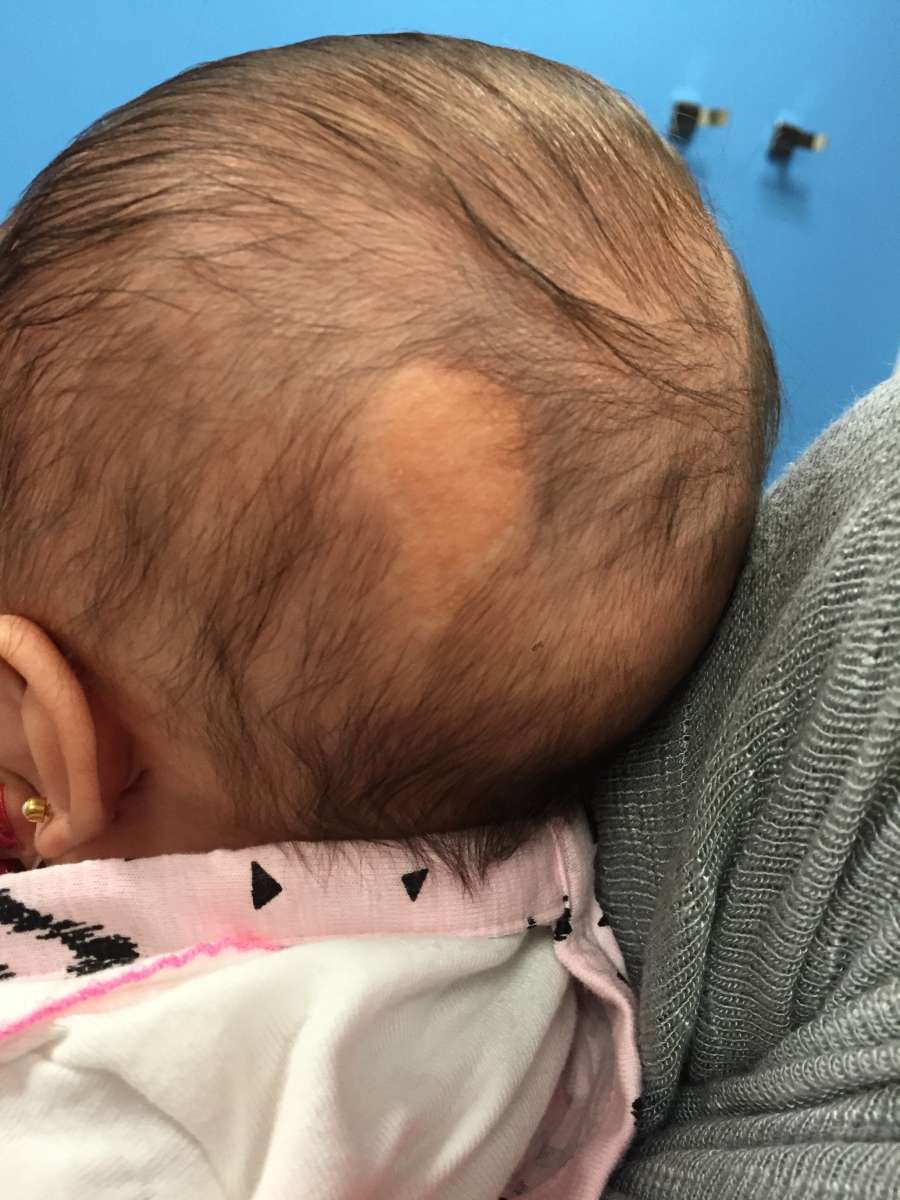The image features a close-up photograph of a baby's head, focusing on the back and side views. The baby has sparse, wispy black hair with a round bald spot on the back left side of the scalp, possibly around the size of a half dollar. The left ear of the baby is visible and adorned with a small pearl earring. The baby is dressed in a white outfit with a pink collar that includes black triangle designs. This outfit appears to have pink outlines or layers over the white fabric. The baby is being held by someone wearing a gray sweater, whose shoulder can be seen on the right side of the image. The background features a blue wall with two small black objects attached to it in the upper right corner.